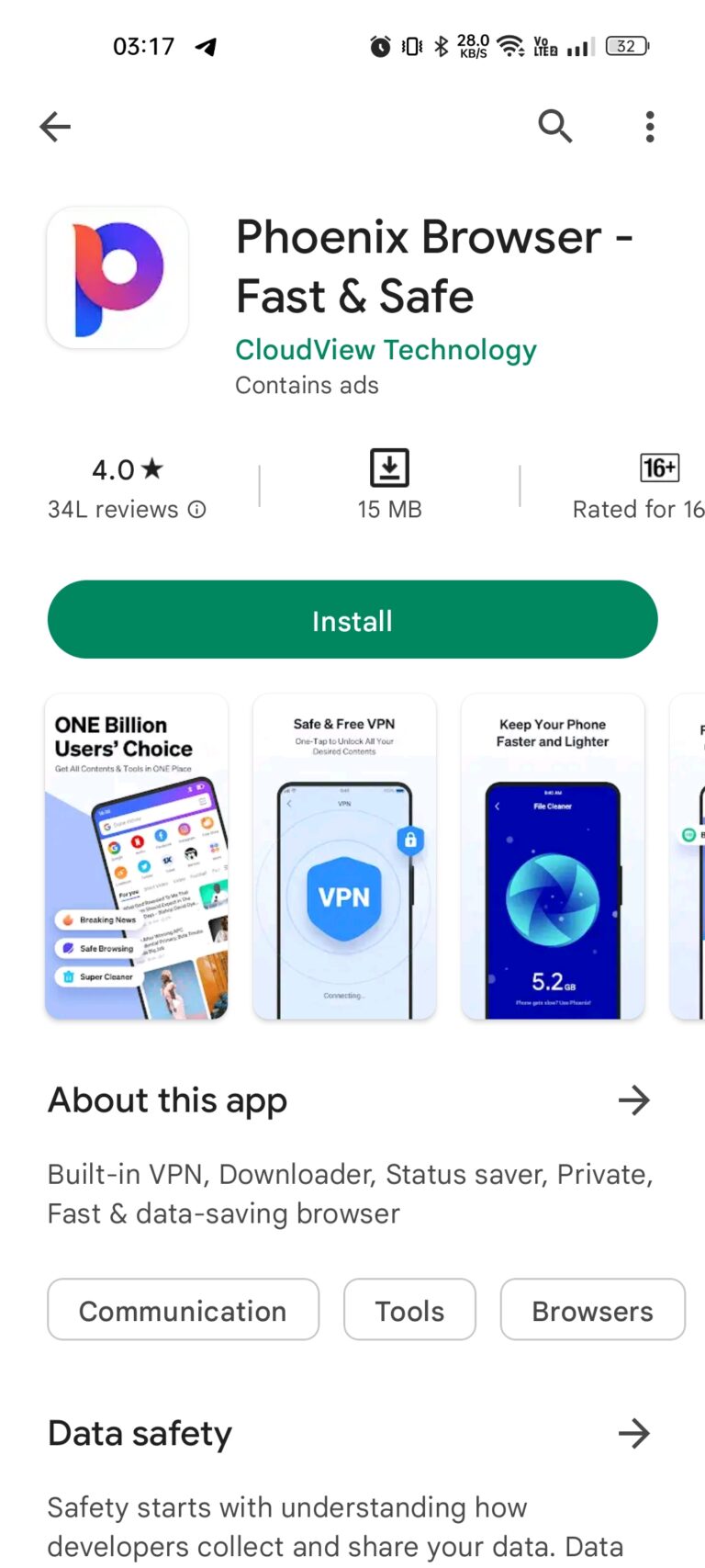A screenshot of an app download page for the "Phoenix Browser - Fast and Safe" app by CloudView Technology. Located at the top, the app's square profile photo displays a red and blue "P" logo. To the right of the logo, the app name is prominently shown in bold, followed by the developer's name "CloudView Technology" in green text. Below the developer's name, a label indicates that the app "Contains ads". Further down, the app's rating is displayed as "4.0" based on "34K reviews".

In the middle section of the screenshot, a download icon is shown alongside the app's size of "15 MB". To the right, there's a "Rated for 16+" label encased in a box. A green "Install" button is prominently placed below this section. 

As you scroll down, thumbnails illustrating the app's key features are displayed. Further down, a section titled "About this app" includes a right-pointing arrow and a brief one-sentence description of the app. Below this, the app is categorized under "Communication Tools" and "Browsers".

At the very bottom of the screenshot, there's a "Data Safety" section to the left with a right-pointing arrow and a message stating, "Safety starts with understanding how developers collect and share your data," with the rest of the text cropped out.